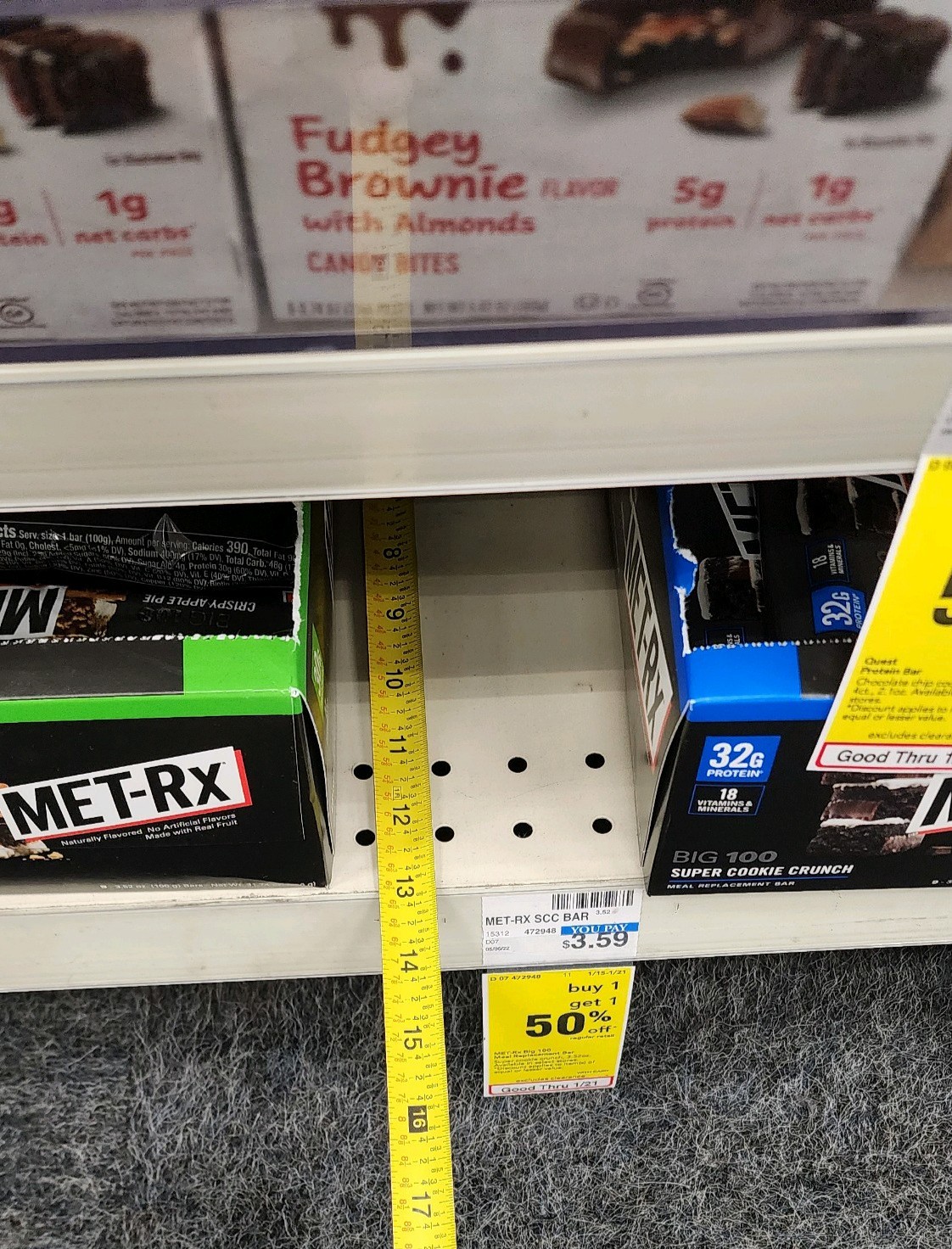In this detailed photograph, we see a retail shelf, likely in a Walgreens or CVS store, meticulously measured for depth with a ruler or measuring tape showing exactly 13 inches. The shelf is stocked with various nutritional bars, including one in a striking black and green box labeled MetRx, and another black bar with blue text indicating 32 grams of protein. Sheltered behind a glass section, there are decadent fudgy brownies studded with almonds. The floor is carpeted in shades of gray and white, adding a muted backdrop. Promotional signage is prominently displayed on the shelf, highlighting a special offer: buy one, get one 50% off.